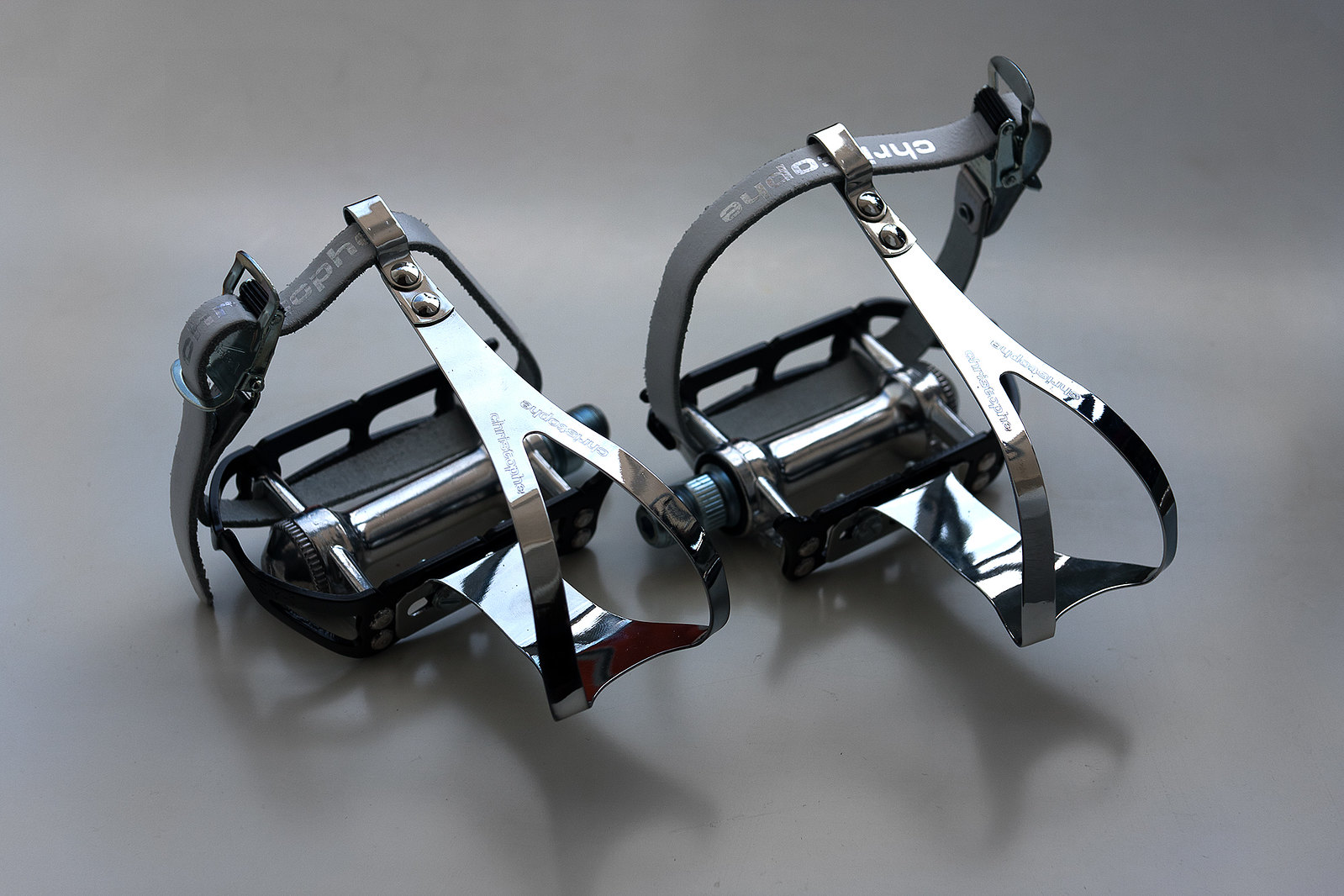The image depicts two bicycle pedals placed on a shiny, gray surface. The pedals, predominantly black and silver, feature straps designed to secure the rider's feet, typically found on racing bikes. The shiny metal of the pedals contrasts with the dark straps, and there are reflective elements hinting at the presence of other colors, such as a touch of red. The binding, which is where the toes slip in and are secured over the shoe, appears new and includes some gray writing on the leather. This detailed composition focuses on the sleek and polished appearance of the pedals, suggesting they are either newly purchased or in the process of being replaced.